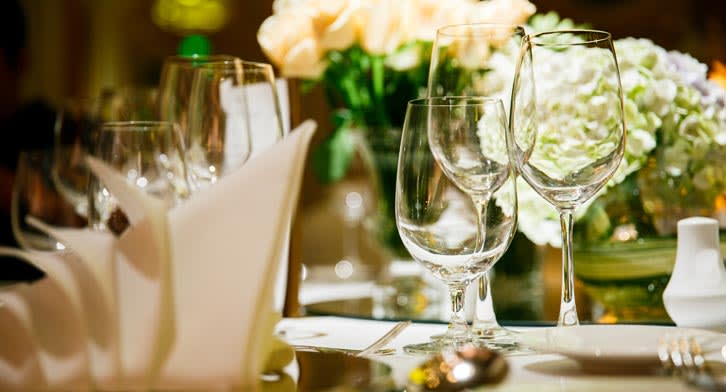This professional, color photograph captures a detailed close-up of an elegantly arranged dinner table. Central to the composition are three empty wine flutes of varying heights. These glasses are positioned prominently in the middle of the table, drawing the eye. To the left, several more wine glasses are seen standing in a row, each uniquely wrapped in white fabric, resembling flowers with the glass stems emerging gracefully. The right side features additional wine glasses, creating a sense of balance and symmetry.

The background is adorned with an arrangement of peach and white flowers, likely roses or sunflowers, in clear glass vases, their delicate hues adding a soft, romantic touch to the scene. The flowers’ green stems are visible, enhancing the natural elegance of the setting. Below, on the table, ornately folded napkins rest in front of the left goblets, complemented by slightly blurred silverware, including a fork and spoon in the foreground, adding to the table’s sophisticated decor.

The table itself is adorned with simple white plates and a solid white, cylindrical salt and pepper shaker, subtly blending into the pristine white tablecloth. Overhead, lights shine down, casting a gentle glow over the entire setting, emphasizing the clarity of the glassware and the freshness of the floral arrangements. This image captures the refined beauty and meticulous detail of a professionally set dinner table, ready for an elegant dining experience.